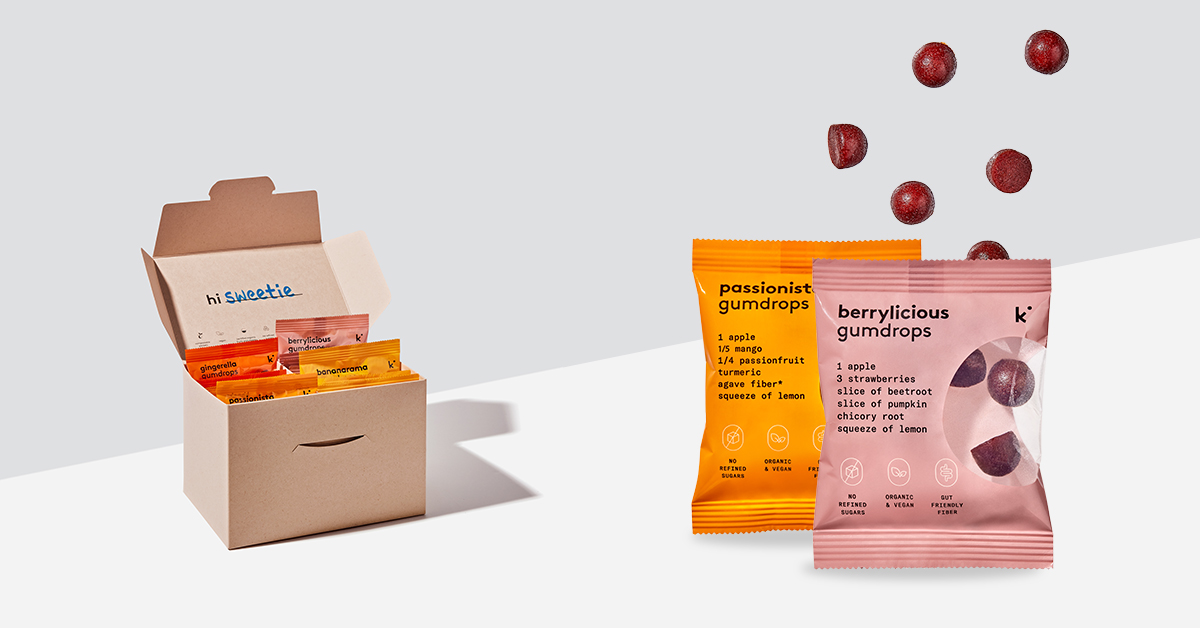This advertisement showcases High Sweetie's Berrylicious and Passionist gumdrops. The vibrant image features a small open box filled with various bags of these gumdrops on the left side. On the right, two bags are prominently displayed, one behind the other. The back bag is orange and partially obscured, while the front one, labeled Passionist Gumdrops, lists ingredients including one apple, one-fifth mango, one-quarter passion fruit, turmeric, agave fiber, and a squeeze of lemon. Next to it, the Berrylicious Gumdrops bag highlights ingredients such as one apple, three strawberries, a slice of beetroot, a slice of pumpkin, chicory root, and a squeeze of lemon. Both bags feature a viewing window on the right to glimpse the colorful gumdrops inside. Scattered across the scene, gumdrops appear to float weightlessly, adding a whimsical touch to the advertisement. The background box also mentions additional flavors, although they remain unreadable.